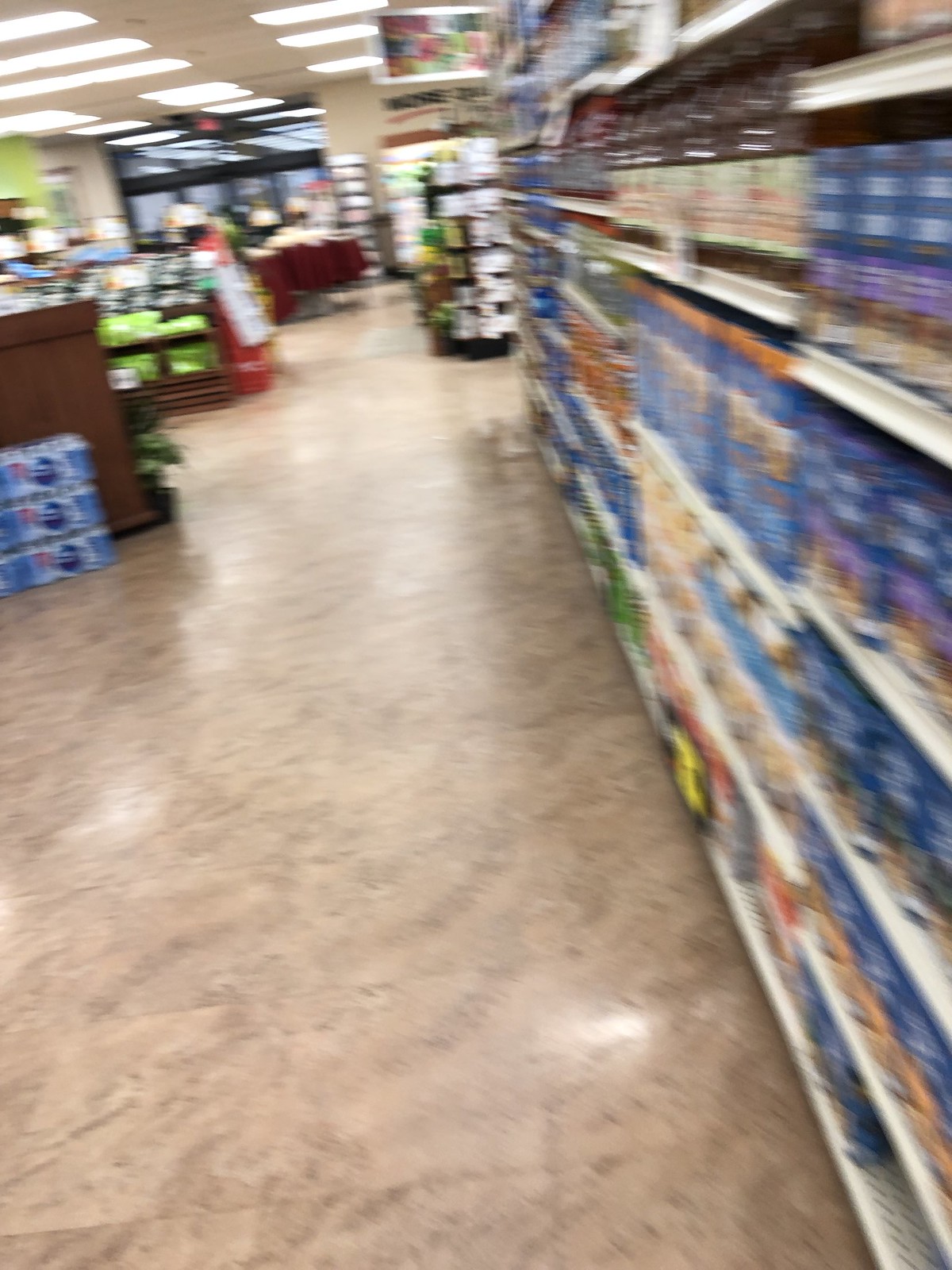The image captures a blurry, slightly tilted view down an aisle of a bustling supermarket. The reflective, shiny floor features a tile pattern with varying shades of brown and beige. On the right side, there are multiple shelves stocked with various boxed and canned goods, including a noticeable section of blue boxed items and bottles with pale yellow labels. Higher up on these shelves, there are possibly jars or bottles of dark red or brown liquid. Across the aisle, a display of stacked Pepsi cartons can be seen. Towards the back of the supermarket, glass doors beneath an exit sign are visible, alongside a green area that might be the produce or deli section. The overhead lighting fixtures are also faintly discernible, highlighting the well-lit atmosphere of the store.